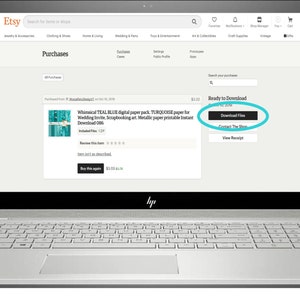The image features an open laptop displaying a personal Etsy customer page. Prominently visible is the Etsy website interface with its familiar layout, including a search bar at the top. Various navigation and menu options are clustered to the right of the search bar and continue below it. The text on the page is mostly unreadable in the image, but the word "Purchases" can be distinctly made out. Adjacent to this are more menu options.

Below this section, there's a visible whimsical teal blue image, accompanied by a brief, unreadable description and additional information. To the right of this teal image, more menu items are listed. One of these buttons, likely a call-to-action such as "Subscribe Now" or "Buy Now," is encircled and highlighted in a teal or blue color, drawing attention to it.

The laptop's keyboard is partially visible at the bottom of the frame, grounding the viewer in the digital and personal workspace setting.